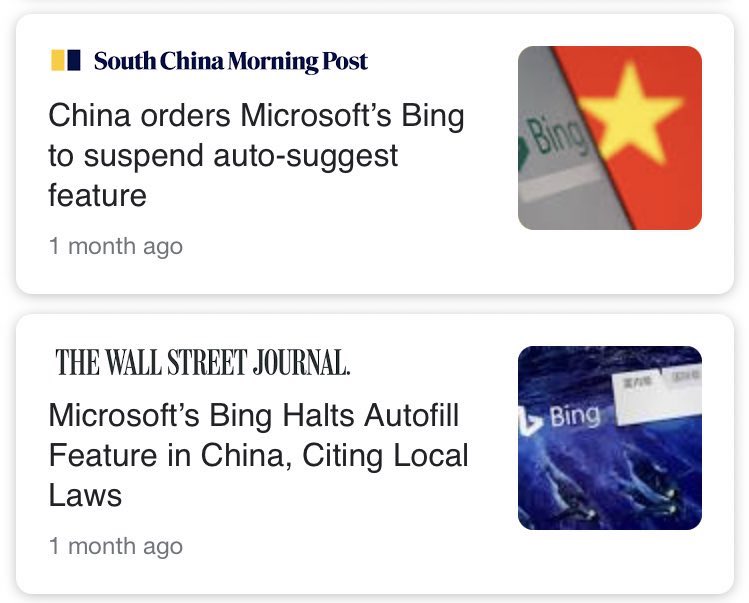This image showcases two distinct newspaper headlines captured in a screenshot. Each headline is enclosed within a rectangular box with rounded corners, and the boxes are stacked vertically in the image.

The first headline, situated at the top, is from the South China Morning Post. This headline features a small yellow and blue square in the upper left corner, serving as a visual branding element. The headline reads, "China orders Microsoft's Bing to suspend auto-suggest feature," highlighting that this news was posted one month ago. To the right of this text, there is an icon divided diagonally: the left side has a gray background with the word "Bing," and the right side has a red background with a yellow star.

The second headline, located at the bottom, is from The Wall Street Journal. It states, "Microsoft's Bing halts autofill feature in China, citing local laws," and this headline was also posted one month ago. Adjacent to this text, on the far right, there is a square image featuring a blue background with the word "Bing" displayed diagonally from the center left. 

Together, these headlines provide a coherent narrative about regulatory actions affecting Microsoft’s Bing search engine in China, presented with distinctive visual branding elements for each publication.